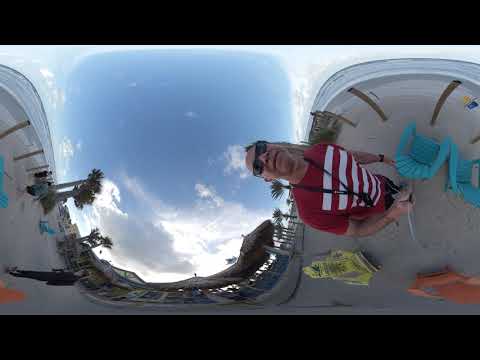The image is a highly distorted, vertically rectangular photograph featuring a man standing on a gray concrete sidewalk, surrounded by a surreal and warped landscape. The picture has black horizontal stripes across the top and bottom, adding to its unusual appearance. The man, a white individual, is sporting black sunglasses, a red and white t-shirt, black shorts, and a watch on his left wrist. He is standing in a side profile, and due to the extreme warping, he appears horizontal on the right side of the image. 

In the background, there are elements of a beach scene with teal beach chairs, palm trees, and pavilions, all made tiny by the distortion. The sky is part cloudy, part clear, and fills a large curved area of the image, resembling a liquid surface pushed and deformed by an invisible glass. This curvature makes the sidewalk appear extremely tall and swooping deeply downwards, creating an almost surreal, dreamlike effect. The entire scene, while recognizable, is rendered almost abstract due to the heavy editing, making it seem simultaneously familiar and bizarre.